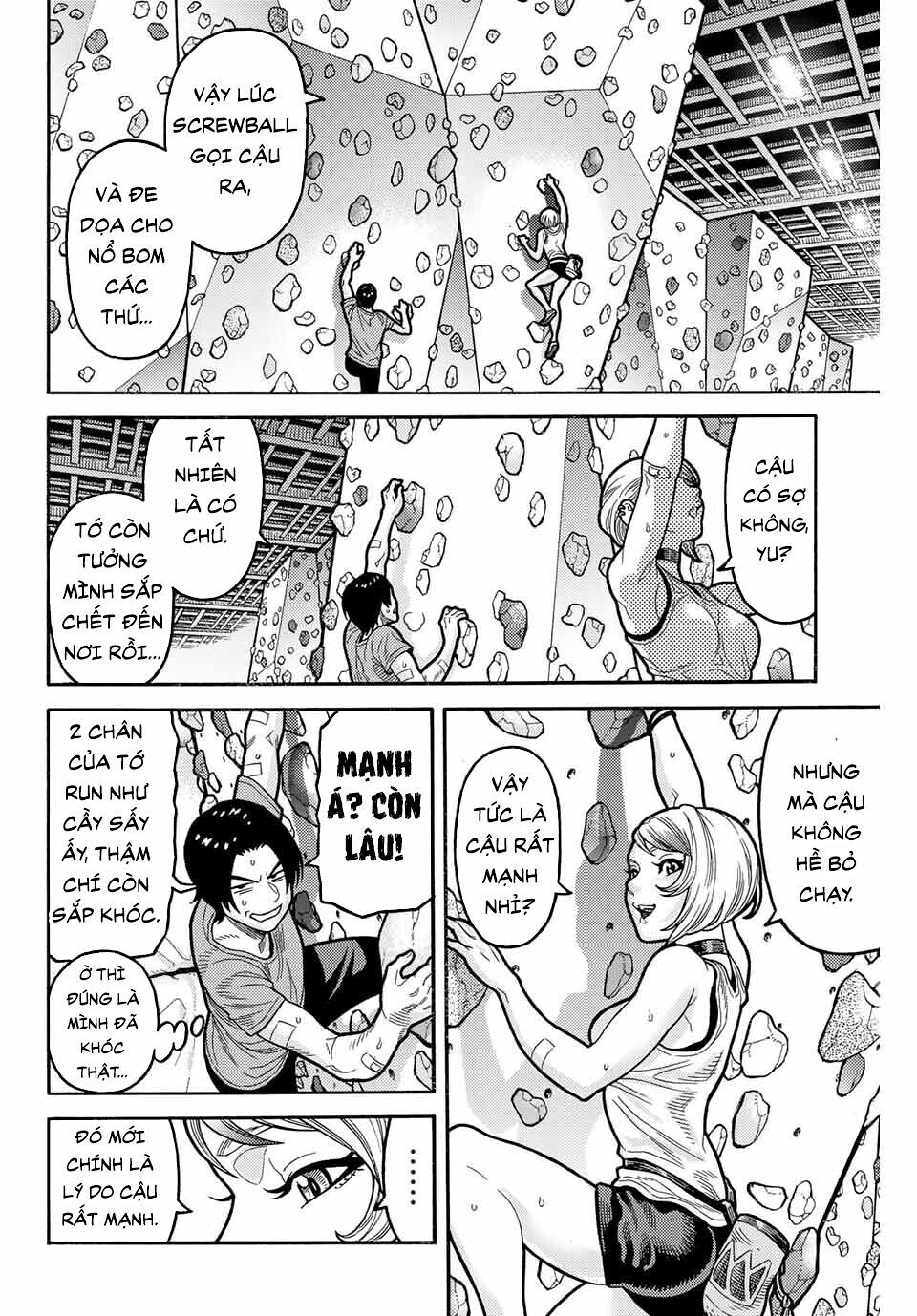The image is a detailed black and white comic strip consisting of five panels, depicting a man and a woman climbing a rock wall together. The top panel is the largest and shows both characters scaling the cliff side, with text in a foreign language that appears to be Japanese. The second panel provides a closer view of the man and woman, clearly illustrating their effort and proximity as they climb side by side. Next, the third panel presents just the man, visibly angry and speaking. The fourth panel focuses on the startled expression of the woman, considered cute by observers, who is also speaking. Finally, the fifth panel, featuring the woman's eye and a portion of her face expressing alarm, is positioned at the bottom left. Each character in the comic is involved in climbing the rock wall while engaged in dialogue throughout the sequence, enhancing the tension and interaction between them.